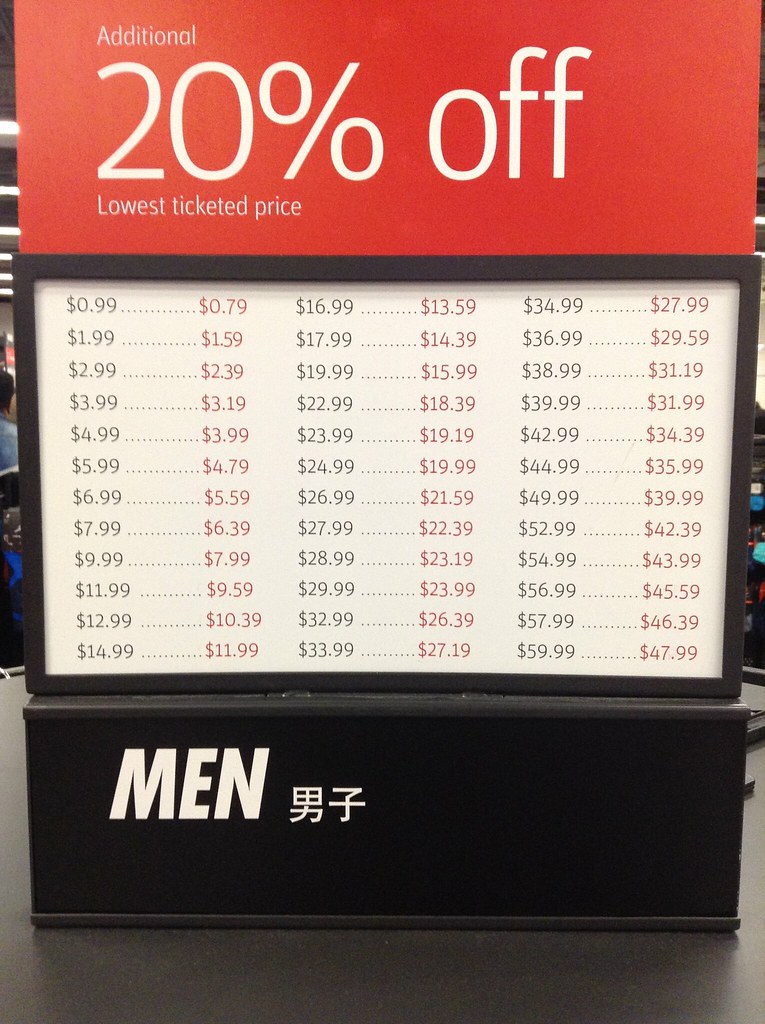**Caption:**
A promotional sign at a department store announces an ongoing sale with an additional 20% off the lowest ticketed price. The sign highlights various discounted prices, starting from 99 cents now reduced to 79 cents, and continuing in increments such as $1.99 to $1.59, $2.99 to $2.39, up to $59.99 now being $47.99. The entire list of price reductions is detailed extensively across the sign.

The sign features a striking design with the majority of the text, including the "additional 20% off lowest ticketed price" statement, in white on a black background. The promotional header for the 20% discount is displayed prominently in white against a red background, ensuring high visibility. At the bottom, the word "Men" is written in white, accompanied by some Asian characters, indicating the section of the store or perhaps the target demographic for the sale. The red and black color scheme of the sign captures attention, and though a few people are visible behind the sign, the specific identity of the store remains indeterminate.